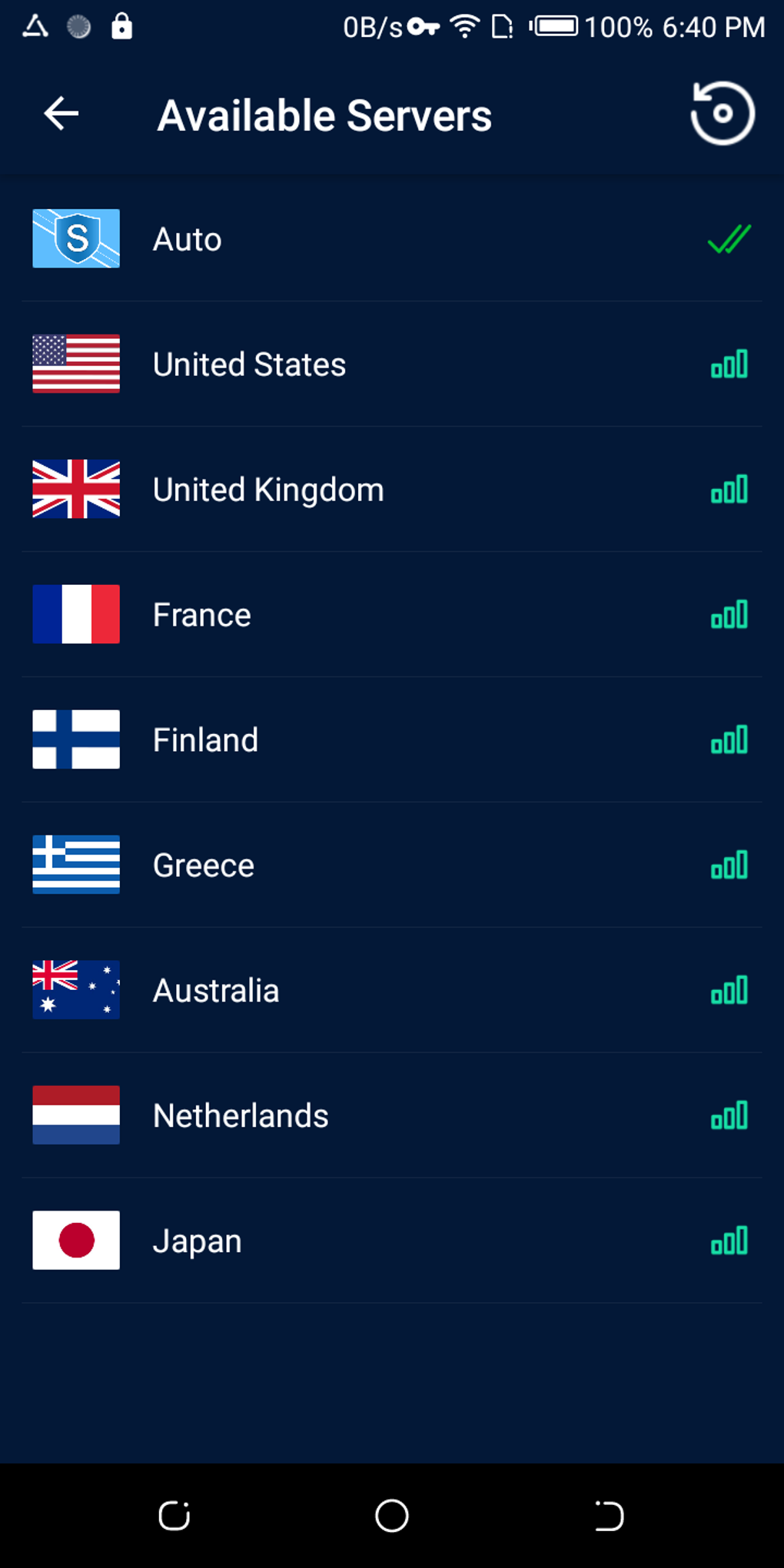The image features an intricate interface with a multitude of icons and symbols. At the top of the triangular layout is a circle and a lock icon. Adjacent to this, there’s an icon representing a Wi-Fi key. The display shows a 100% battery life indication with a capacity of 640 mAh. Below are additional indicators, including a rotating circle symbolizing the third available service.

The visual elements further include a blue square and a shield with an 'S,' signifying an auto feature. There are also double green check marks confirming a positive status. Country indicators are prominently displayed: the United States with partially filled signal bars, the United Kingdom with a blue, white, and red pattern, Finland with a white and blue bar, and Greece with alternating blue and white bars.

The backdrop of the image is a neutral grey. Additional country flags appearing include Australia depicted in blue with not fully filled signal bars, the Netherlands in red, white, and blue, and Japan represented by a black bar. A red dot alongside the Wi-Fi symbol denotes some form of status indicator, and lastly, another rotating circle is present, potentially indicating loading or processing.